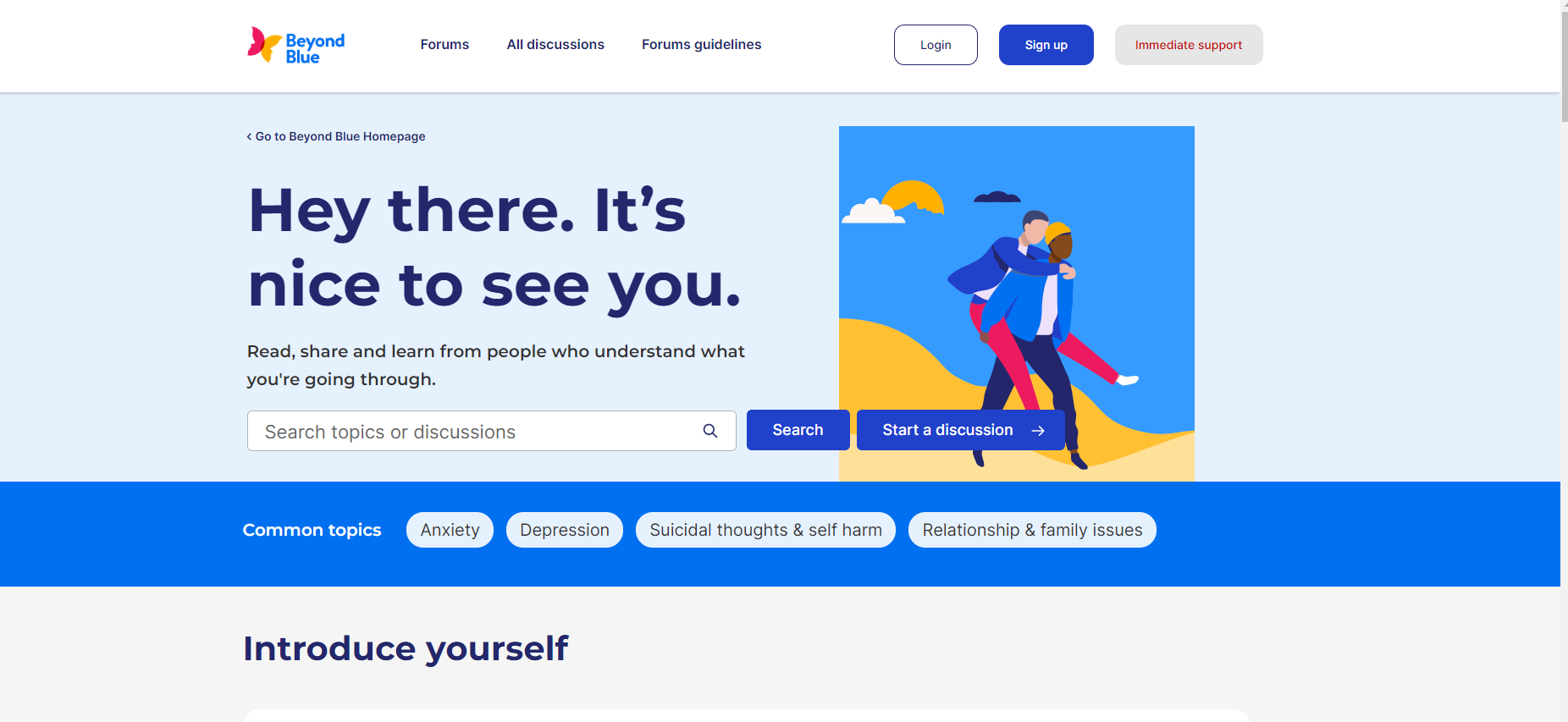Screenshot of the Beyond Blue homepage. On the top left, "Beyond Blue" is prominently displayed, accompanied by links labeled "Forums," "All Discussions," and "Forum Guidelines." On the top right, there are options to "Login," "Sign Up," and a highlighted "Immediate Support" button. At the center of the page, a welcoming message reads, "Hey there, it's nice to see you." Directly below, a helpful tagline states, "Read, share, and learn from people who understand what you're going through." The middle section features a search bar with the placeholder text "Search topics or discussions" and a blue "Search" button. Next to the search bar, a "Start a Discussion" button is available for users to initiate new conversations.